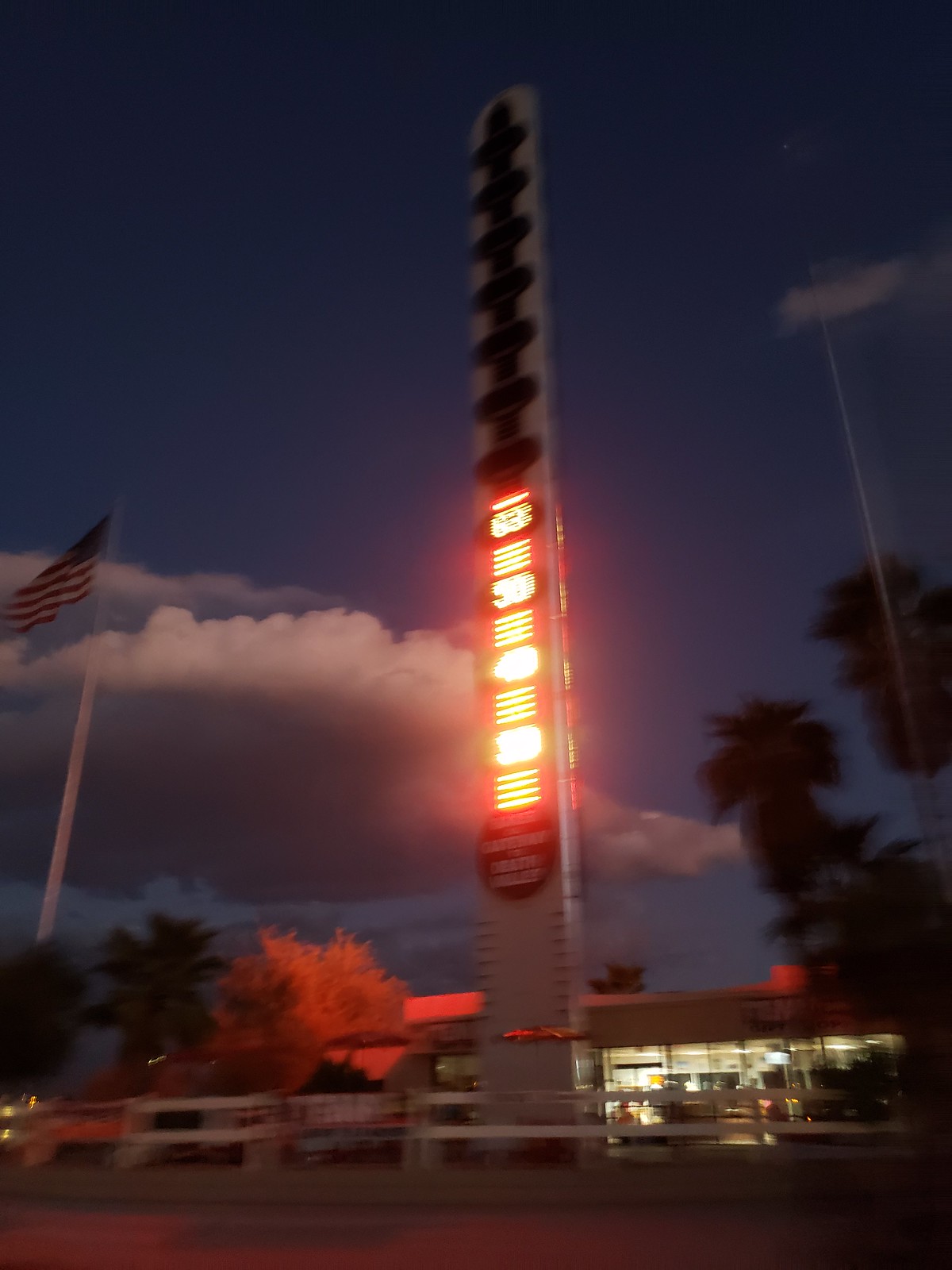In this nighttime image, we observe a blurred scene likely captured in motion, possibly by someone driving or walking by. The central focus is a tall, slender gray tower or pillar with a series of illuminated numbers in red neon, displaying 30, 40, 50, and 63 as it ascends. Above these, the lighting fades, leaving the upper section unlit. Angled lines between oval shapes run the length of the pillar. The sky is dark, featuring large white fluffy clouds. In the left-hand corner, an American flag on a white flagpole waves in the wind. Beneath the flag and clouds, green trees, with one seemingly reflecting the tower's light, add to the scene. A single-story building, its lights on, stands in the middle of the photo, hinting at a roadside store. Palm trees are also visible on the left side of the image. The overall setting suggests a road or street, providing a glimpse into a vibrant nighttime landscape.